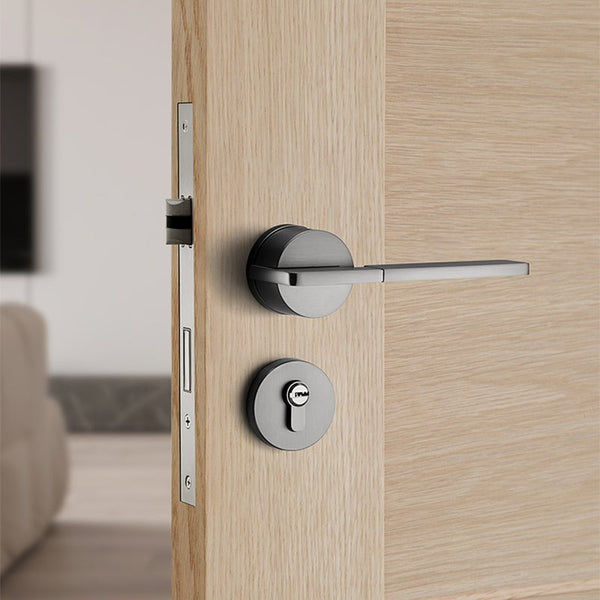The image depicts a close-up view of an open, light brown wooden door with modern hardware. The door features a horizontal, black handle at the top, extending outward like a lever that's easy to push down. Directly below the handle is a circular, black key lock. A long, narrow rectangular silver plate is visible on the side of the door, showing the metallic part of the latch that extends into the doorway. The background of the image is blurred, revealing what appears to be a white wall adorned with a partial view of a black TV monitor hanging on it. There is a gray trim around the lower part of the wall, and the flooring seems to be a gray laminate or hardwood. The bottom left corner of the image catches the edge of what looks like a couch, contributing additional context to the room's setting.